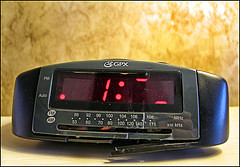The image depicts a vintage alarm clock with a distinct AM/FM radio dial. This particular model has a unique rectangular shape with a domed top. To tune into radio stations, one had to manually slide a control along the dial. The device likely possessed subpar speakers, characteristic of its era. Notably, the LED display for the time appears to be malfunctioning, showing only one colon and two horizontal lines above and below it. The left side of the display features indicators for AM and PM, which were essential to set correctly to avoid the alarm going off at the wrong time, like 8 PM instead of 8 AM.